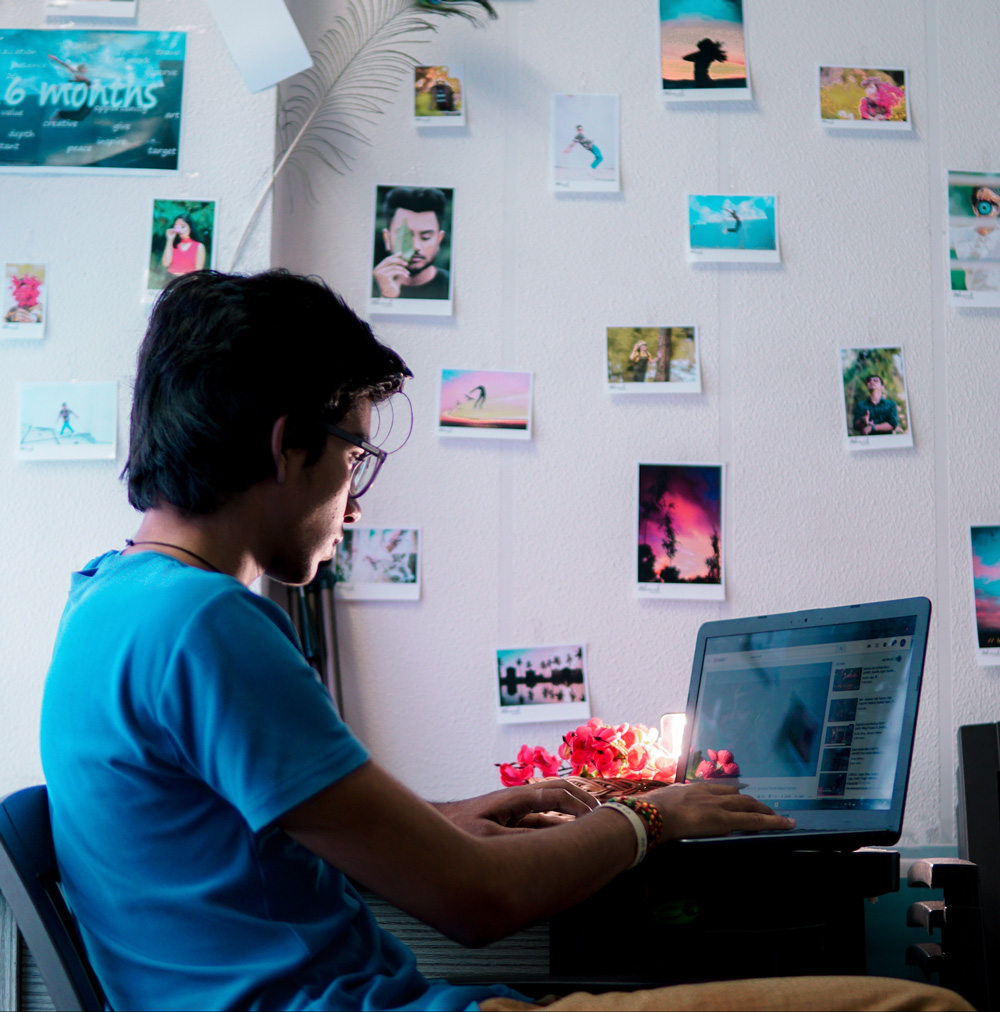A young man with short black hair is deeply engrossed in his laptop while sitting at a desk in a room. He is dressed in a blue short-sleeved t-shirt and possibly jeans or brown pants. The laptop screen displays a YouTube page. The white-painted wall behind him serves as a creative backdrop, adorned with various printed photographs reminiscent of Instagram posts, attached at irregular intervals and heights. 

In the top left corner of the wall, a poster with the words "six months" is partially visible. Below this poster, three photos are displayed. A striking peacock feather extends from just above the young man's head, reaching beyond the frame of the image. To his right, a cluster of 14 photos is affixed to the wall, creating a vibrant collage.

On the desk, behind the laptop, there is a light source and what appears to be a bouquet of flowers. The young man accessorizes with bracelets on his right wrist and a necklace, likely made of leather, around his neck.